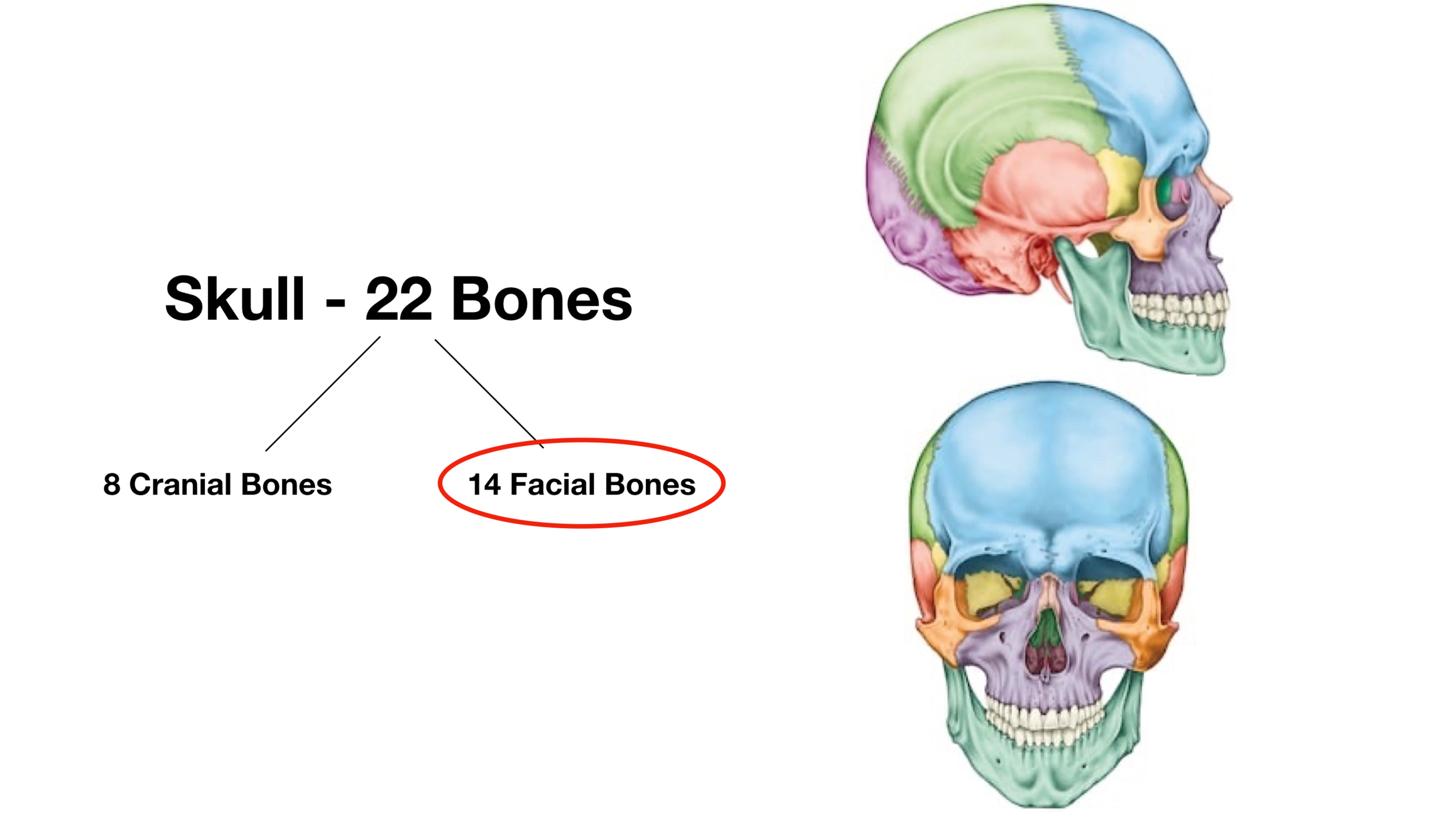The rectangular image, likely used for educational purposes, features a detailed anatomical illustration of a human skull with multiple views and accompanying text. The skull is depicted in two positions: the top right side displays a profile view facing right, while the bottom right shows a frontal view. The skull is color-coded to distinguish various bones, with sections in blue, green, purple, red, and orange, and the teeth are white.

On the left side of the image, large black text reads "Skull - 22 Bones," with additional black lines and text providing further information. A line pointing downward to the left indicates "8 Cranial Bones," and another line pointing downward to the right, encircled by a red oval, notes "14 Facial Bones." The text and lines help to pinpoint and categorize the different parts of the skull displayed in the two colored illustrations on the right. The overall image lacks a definitive border, blending into the white background of the screen.